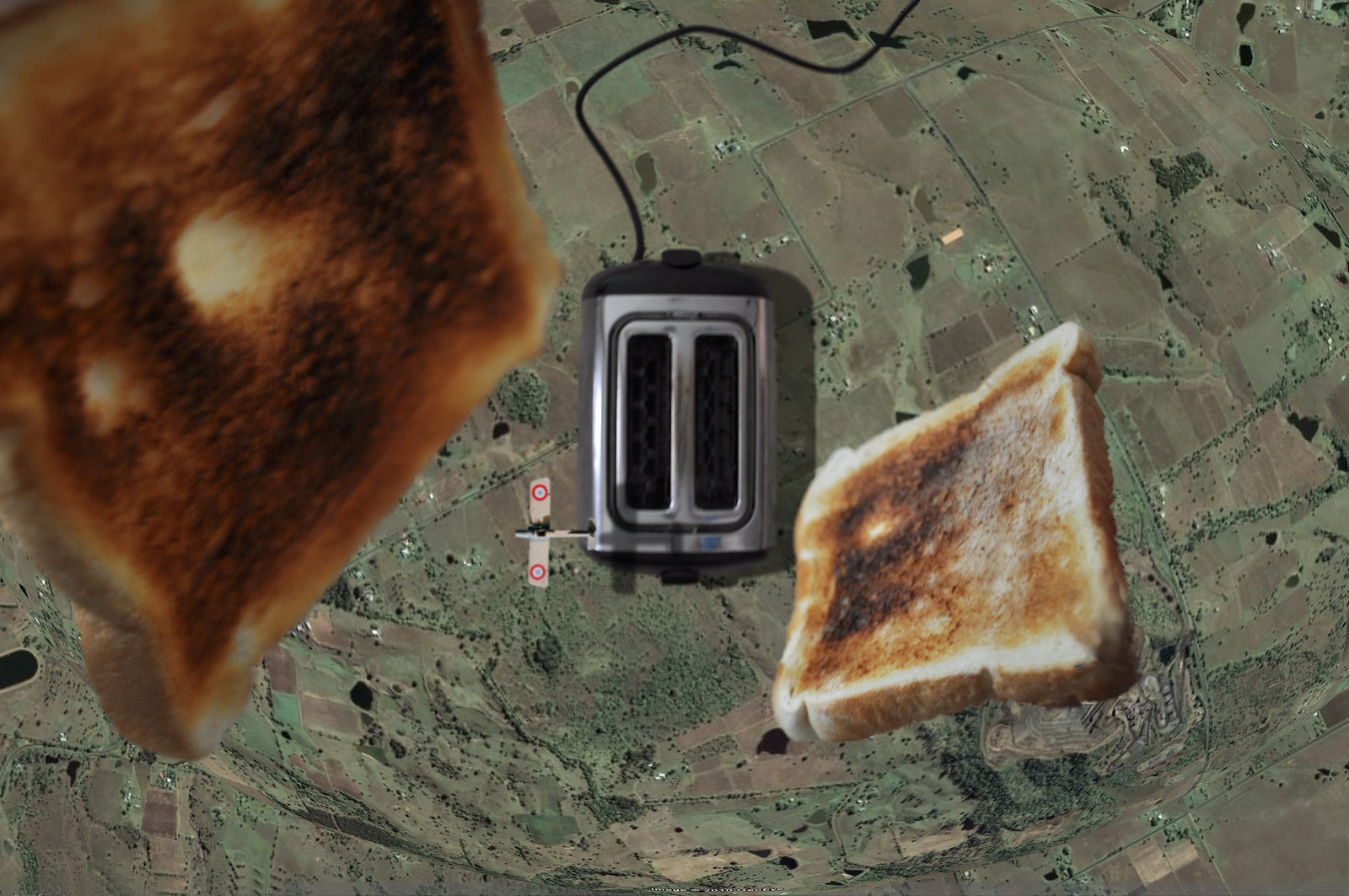This surrealistic aerial photograph captures a shiny silver toaster in a peculiar mid-air setting, as if viewed from a considerable height. The scene resembles a green and gray earthen map or farmland, evoking a sense of gazing at ground features from 10,000 feet up. Centered in the image, the toaster is depicted with a long black power cord trailing behind it. Two pieces of toast are seen flying outward and upward from the toaster, adding a dynamic and whimsical element to the shot. The toast slices exhibit varying degrees of browning, with one piece, located in the upper right corner, appearing more darkened and partially cut off at the top. The other, positioned left of center, shows inconsistent toasting, with a particularly darker center.

Adding to the eccentricity, the bottom right corner features a miniature tan airplane, detailed with red, white, and blue bullseyes on its wings, suggestive of a World War II era design. The plane casts a shadow on the toaster, further blurring the lines between reality and artistry in this AI-generated image. Overall, the photograph conveys an imaginative narrative, akin to a toaster and its toast skydiving over a vast, miniature landscape.